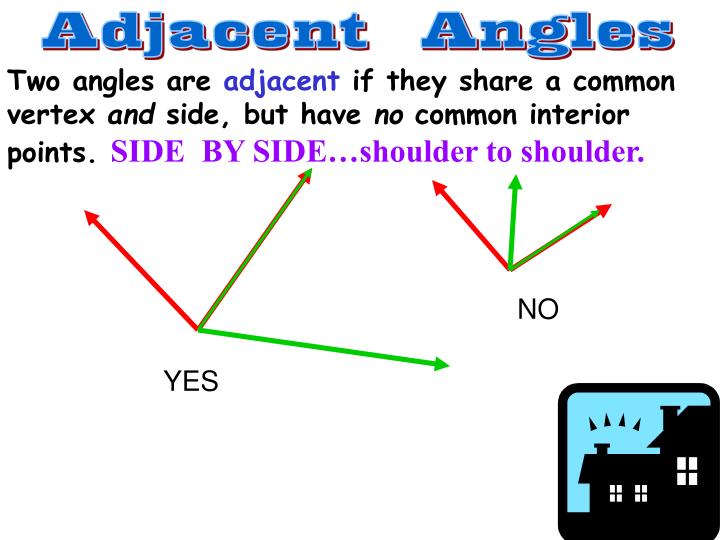The image explains the concept of adjacent angles on a white background. At the top, bold blue letters state "Adjacent Angles." Below that, in a mix of black and purple Comic Sans font, it reads, "Two angles are adjacent if they share a common vertex and side but have no common interior points." The phrase "side by side, shoulder to shoulder" is emphasized in purple. 

Beneath this text are graphical representations: on the left, a red arrow converges with two green arrows at a common vertex, labeled "YES" in capital letters. To the right, smaller red and green arrows intersect but do not share a common side, labeled "NO" in capital letters. 

In the bottom right corner, there's a logo of a black house with lit windows set against a blue sky background.